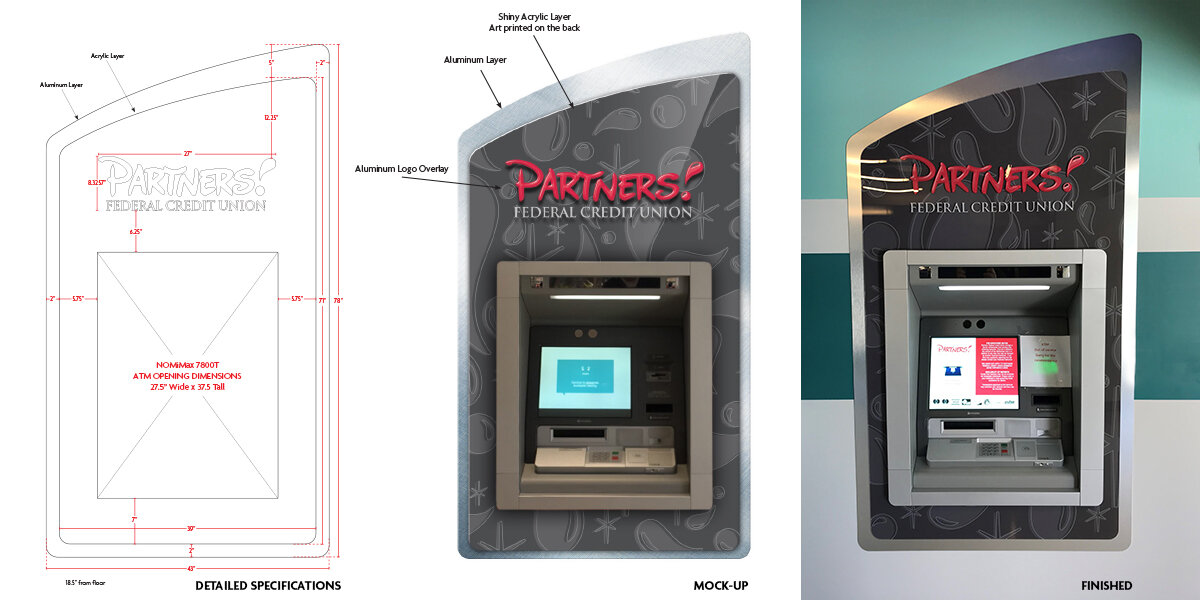This image features a detailed progression of an ATM design in three stages from left to right. On the left side, a black and white schematic displays the precise dimensions and construction specifics, outlined with red and grey lines, indicating the detailed specifications. The central image showcases a more complete rendering or mock-up of the ATM, with components like a screen, keypad, and labeled elements. The top center of the ATM is marked with "Partners" in red followed by "Federal Credit Union" in white, indicating the branding. The rightmost image reveals the finished product, now fully assembled and mounted in a wall. The final ATM model features a silver outline, various functional elements such as lights, a touchpad, money input/output mechanisms, and detailed labeling indicating its aluminum and shiny layers, thus illustrating the transition from conceptual blueprint to finalized installation.